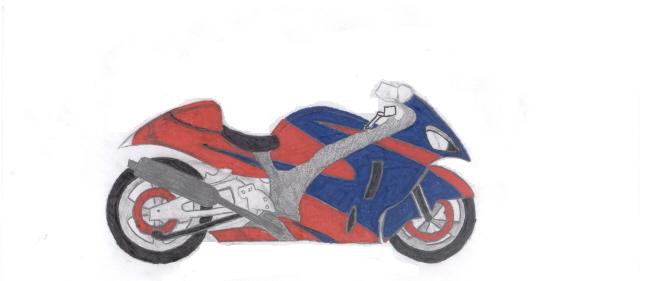This side-view illustration showcases a striking motorcycle design. The motorcycle's body predominantly features a vibrant red color, accentuated by horizontal blue stripes on the rear section. The handlebars are positioned on the right side of the bike. The front part of the motorcycle, extending from the seat towards the wheel, is adorned with a prominent blue patch that culminates in a sizable blue square near the wheel, resembling a bag in shape and intersected by two elongated blue lines running horizontally.

Adding to the visual intricacy, a gray patch is angled and stretches across the motorcycle's center, providing a dynamic contrast to the red and blue hues. The wheels boast red rims coupled with silver spokes and are equipped with black tires. Completing the detailed design, a gray muffler is situated just above the rear tire, contributing to the motorcycle's sleek and polished look.